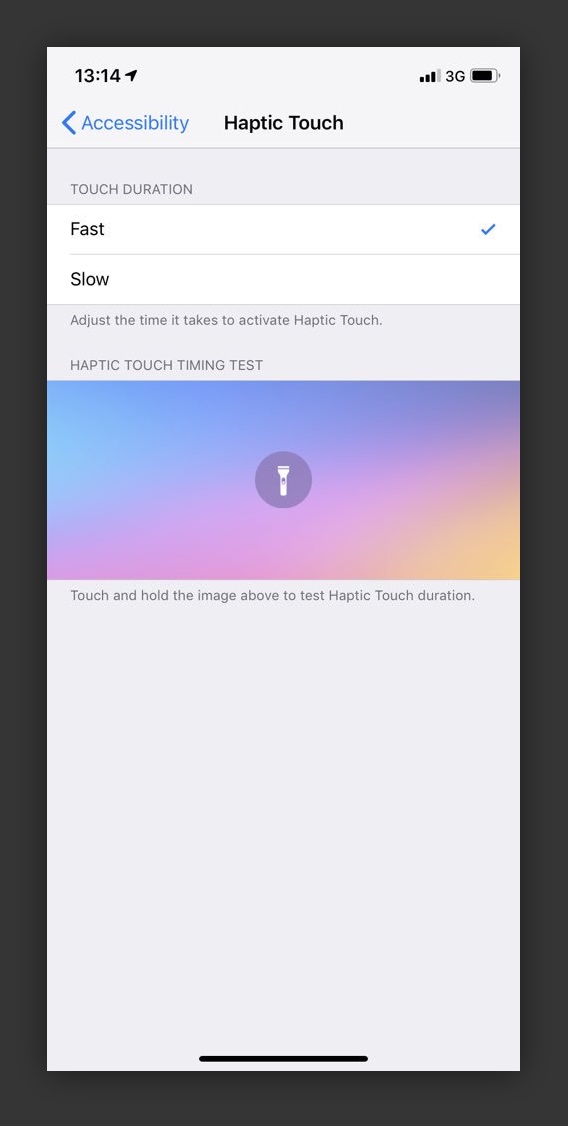This image is a detailed screenshot from an iPhone, set against a dark gray border that might be a design choice to simulate an iPad frame. The screenshot displays an iOS device's screen with a white background. The device’s status bar shows a nearly full battery, a 3G network connection with three out of four signal bars, and a time of 1:14 PM (13:14 in 24-hour format).

The screenshot captures the 'Accessibility' section of the device's settings, evident from the word “Accessibility” in the top left corner, accompanied by a backward-pointing arrow. The focus is on the 'Haptic Touch' settings within the 'Accessibility' menu. Below the title “Haptic Touch,” users can adjust the touch duration, with options for either fast or slow touch response. The currently selected option, 'Fast,' is marked with a blue checkmark.